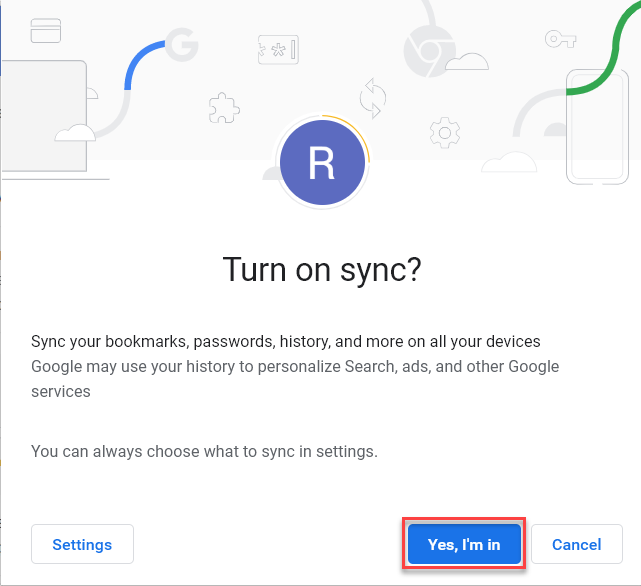The image appears to be a screenshot from the Google Chrome website, featuring a promotional prompt to enable synchronization of user data. The background is a clean white and gray gradient. To the left, there is an illustration of a computer with a gray line extending from it, followed by a gray "G" and a blue dash. Further right, there's a small circle with a squiggly line connected to a ticket stub icon and two arrows. Next to these elements is the Google Chrome logo. On the far right, a clipart image of a phone is depicted with a green squiggle emanating from it.

Beneath this assortment of graphics, there is a bold text header in black reading, "Turn on sync?" This is followed by explanatory text stating, "Sync your bookmarks, passwords, history, and more on all your devices. Google may use your history to personalize search ads and other Google services. You can always choose what to sync in settings." Below this description, three buttons are displayed: a blue button labeled "Settings," a blue button on the right side that says "Yes, I'm in," and a white button with blue text that says "Cancel." The prompt is clearly encouraging the user to activate synchronization of their data across devices using Google services.